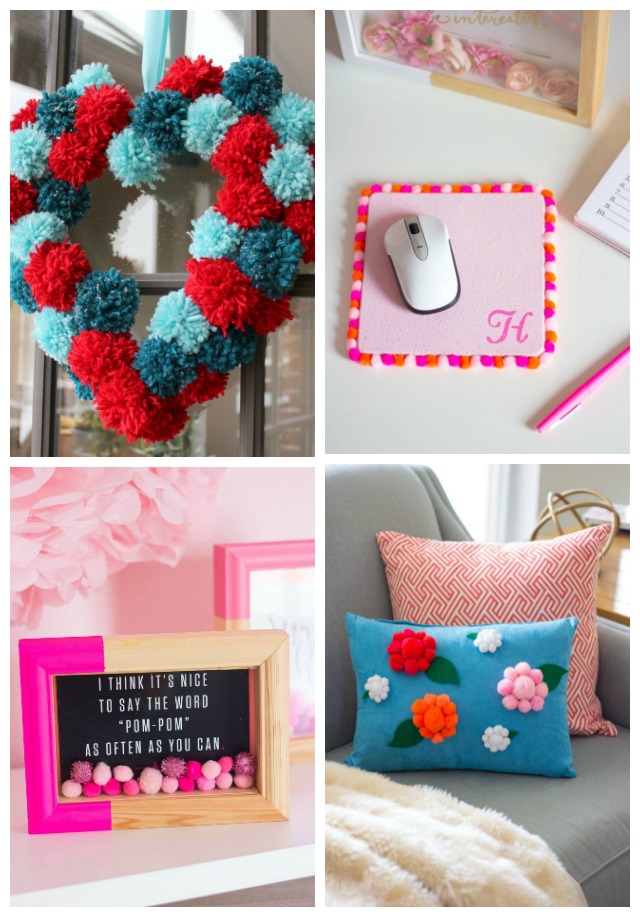This image is a four-quadrant panel showcasing various craft and home decor items, each rich in detail and creativity. 

In the upper left quadrant, there's a heart-shaped wreath crafted from vibrant red, light blue, and dark blue fuzzy balls. This wreath is intricately hung on a glass paneled door using a light blue silk ribbon, adding a whimsical touch against the backdrop of the window.

In the upper right quadrant, a cozy workspace is depicted. A light pink, handmade mouse pad adorned with bright pink, light pink, and orange pom-poms along its borders features a white mouse on top. The mouse pad also has a cursive "H" in the bottom right corner. It's set atop a white desk, which also holds a golden-white floral frame, a notepad, and a pink pen.

The bottom left quadrant showcases a charming piece of framed artwork. The frame itself is partially painted bright pink, contrasting with its natural wood finish. Inside, it reads, "I think it's nice to say the word pom-pom as often as you can," surrounded by small pink and fuchsia pom-poms. Behind this frame is another with pink flowers, adding to the crafty theme.

Finally, the bottom right quadrant captures a cozy gray couch adorned with a white fluffy throw blanket and two decorative pillows. The front pillow is a blue one embellished with red, pink, orange, and white 3D pom-pom flowers, complete with green leaves, giving a textured, handmade feel. The pillow behind it displays a red and white geometric pattern, adding a modern contrast.

Overall, the image is a delightful collage of crafts and home decor, emphasizing the use of colorful pom-poms and cozy materials.